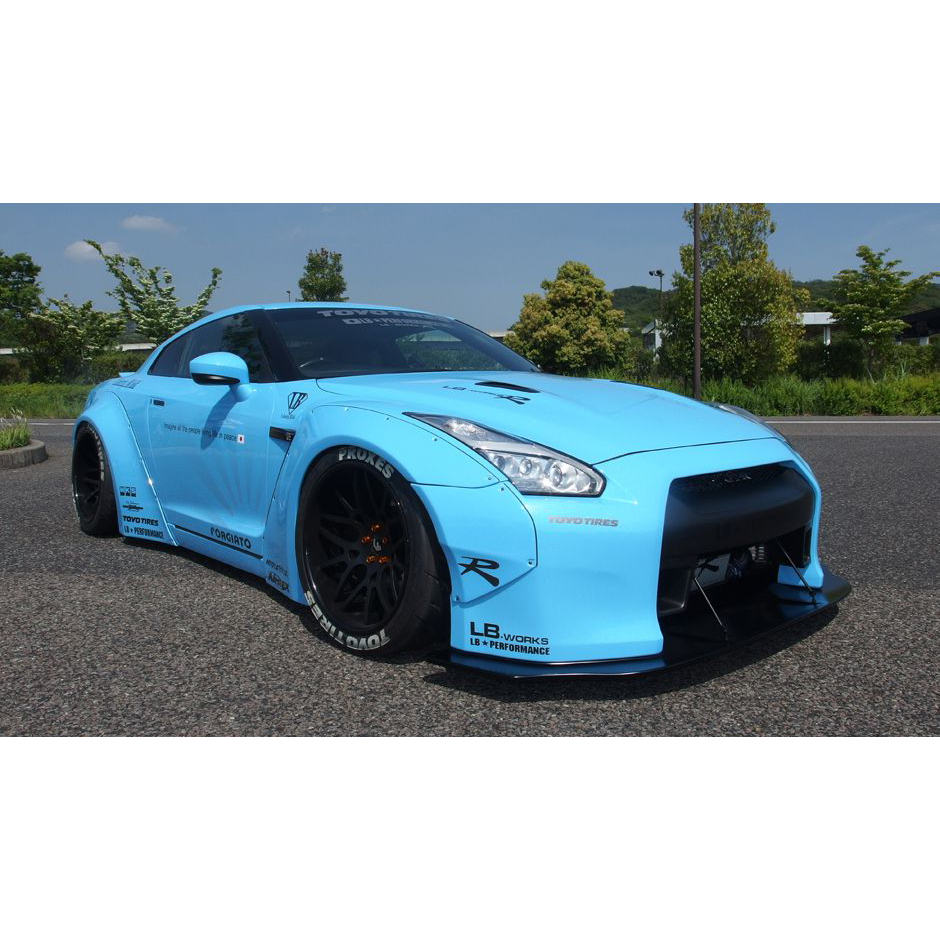This is a detailed photograph of a sky blue race car, designed in the style of a NASCAR, parked on a freshly paved, gray asphalt surface possibly resembling a parking lot. In the background, light green trees give a lush, summery feel under a clear blue sky dotted with a few white clouds. The two-door race car is equipped with large black racing tires and a distinctive black bumper that includes a guard instead of a typical grille. The minimal black writing on the car hints at sponsorships or branding, mentioning something about tires and LB works. The scene suggests a bright day, providing vibrant, well-lit surroundings that highlight the sleek, flat-to-the-ground design of the sports car.